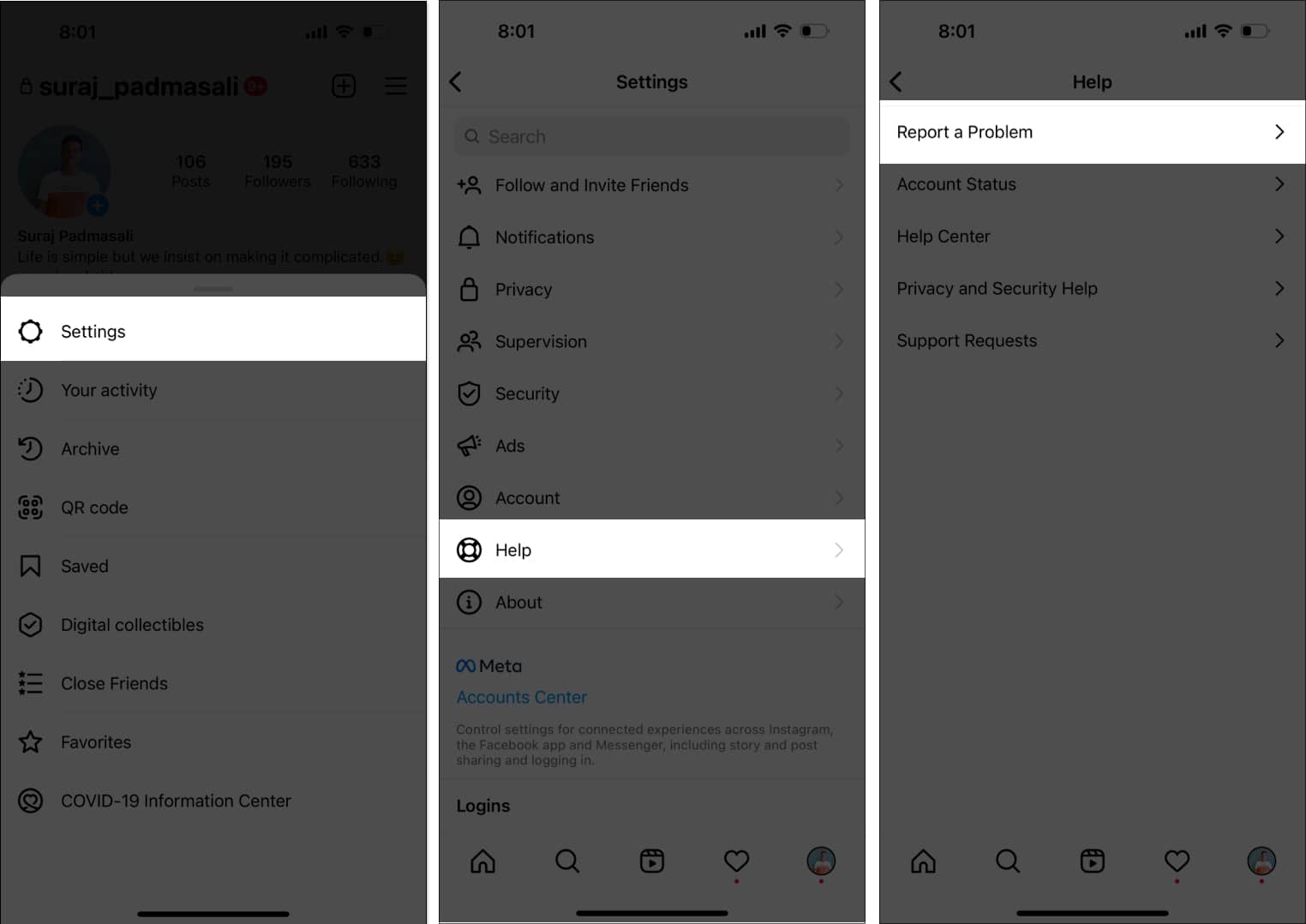The image is a collage of three screenshots, arranged side-by-side in a vertical format. Each screenshot is longer top-to-bottom than side-to-side. The backdrop is a hazy gray, with a prominent white pop-up window indicating user interaction.

**Details of Each Screenshot:**
1. **Top Left Corner:**
   - All three screenshots display the time "8:01."
   - Wi-Fi and internet signals are full.
   - The battery is approximately 25% full.

2. **Left Screenshot:**
   - Shows the main screen with profile details of a user named "Siraj_Padmasali."
   - A slightly blurry profile picture is visible.
   - Below the profile picture, it states:
     - "106 posts"
     - "195 followers"
     - "633 following"
   - The bio reads, "life is simple but we must insist on making it complicated :)"
   - A menu pop-up with several options lights up the "Settings" icon and text.

3. **Middle Screenshot:**
   - The title at the top reads "Settings."
   - A search bar is present underneath the title.
   - Nine clickable options are listed; the "Help" option, second from the bottom, is highlighted in white.

4. **Right Screenshot:**
   - The title at the top reads "Help."
   - Lists five options for user assistance.
   - The first option, "Report a problem," is highlighted in white while the others are light gray.

This detailed caption describes the visual elements and functionalities showcased within the combined screenshots, providing a comprehensive understanding of the image's context.